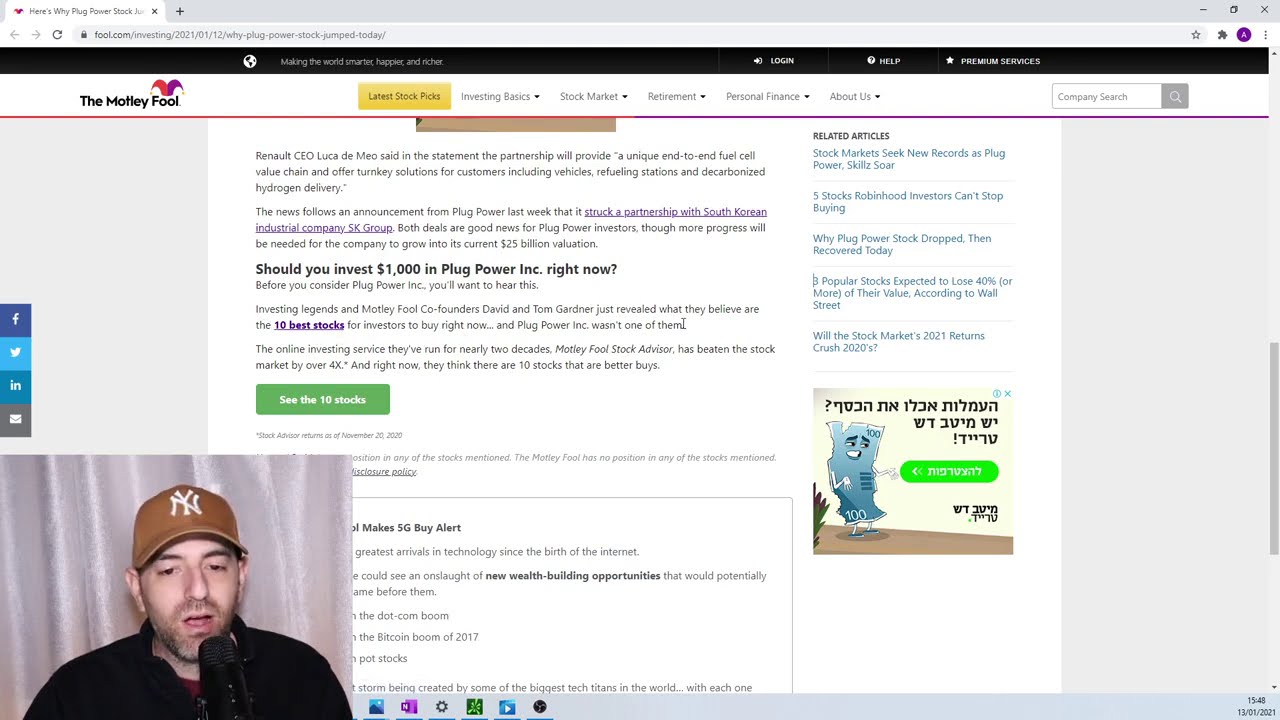The image is a detailed screenshot of a web page from The Motley Fool website, specifically addressing an article titled "Why Plug Power Stock Jumped Today." The article discusses investment opportunities associated with Plug Power Inc. and features typical elements of The Motley Fool's style, including sections like "Should you invest $1,000 in Plug Power Inc. right now?", related articles, advertisements, and social media icons like Facebook, LinkedIn, and Twitter. The webpage also features navigation bars at the top, listing sections such as Investing, Banks, Stock Market, Retirement, Personal Finance, and About Us, with a distinctive jester hat logo of The Motley Fool. In the lower left corner of the screenshot, a man appears to be commenting on the content. He wears a brown New York Yankees baseball cap and a black button-up shirt, has stubble, and is speaking into a microphone while standing in front of a white or off-white curtain. This inset image suggests he is likely streaming a video commentary or conducting a presentation via a platform like Microsoft Teams or Zoom, discussing the webpage's investment topic in detail.